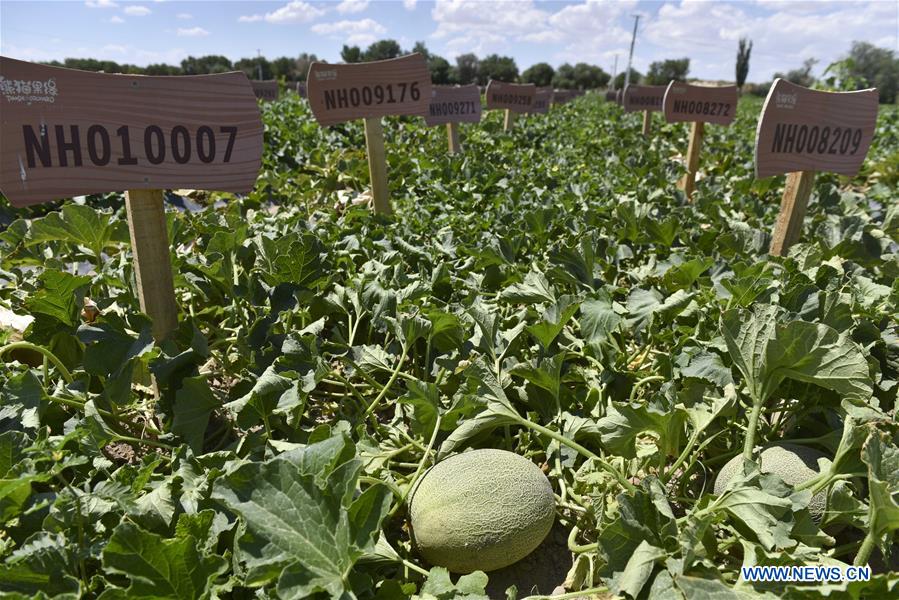This close-up outdoor photograph showcases a lush, green vegetation patch—likely a melon or pumpkin field—featuring large, oval-shaped produce such as melons, with detailed veining on the thick green leaves. In the center-bottom of the image lies a not-quite-ripe melon on its side, while another melon is partially visible in the bottom-right corner. The foreground is dotted with wooden signs—each composed of a vertical post attached to a flat piece, bearing numbers and letters. The signs' engravings include sequences like NH010007, NH008209, and NH09176, marking different sections or plants in the patch. The signs are neatly aligned in two straight rows. The background reveals a tree line with vibrant green leaves against a light blue sky filled with fluffy clouds. In the bottom-right corner of the image, a website—www.news.cn—is displayed in blue with a white outline.